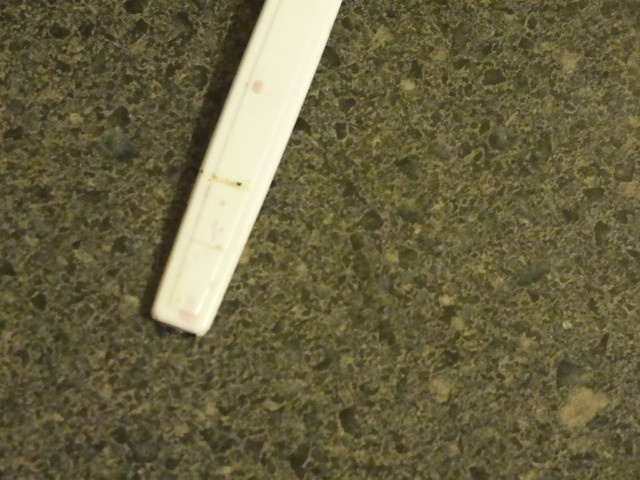A close-up, color photograph taken indoors reveals a surface that closely resembles a granite countertop, characterized by its intricate patterns of brown and green. Positioned slightly off-center to the left, there is a partially visible object that dominates the frame. This object, with a cylindrical yet somewhat rectangular shape, appears to be a white thermometer. The photograph captures the backend of the thermometer, seen from an upside-down perspective. Visible signs of aging and use are evident, with portions of the white surface showing spots of dirt and a yellowing discoloration. A shadow extends from the object towards the left and beneath it, adding depth to the image.